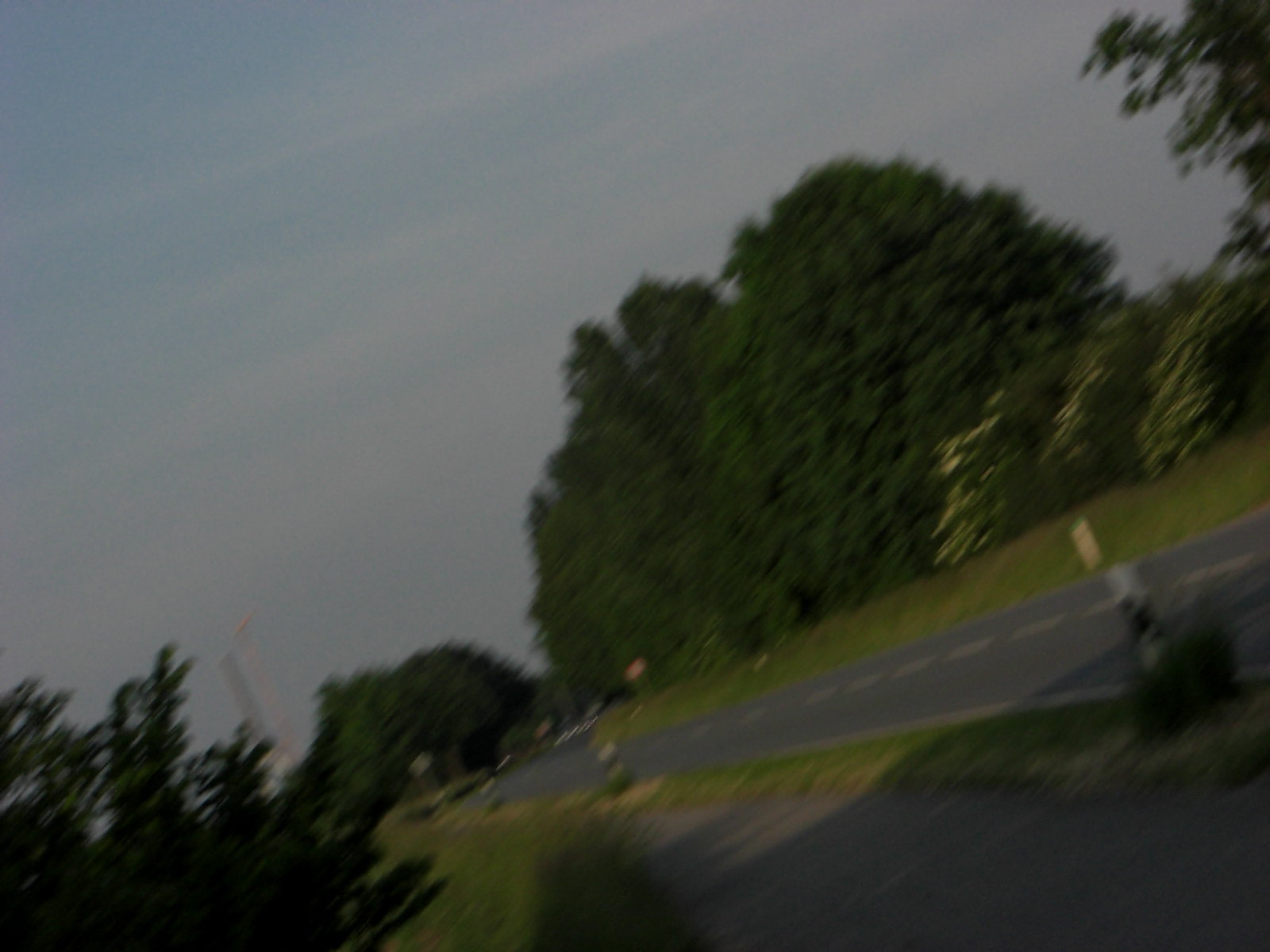This photograph, taken outdoors, depicts a dark and very blurry scene. The image shows a two-lane road that runs from the right-hand side and curves into the background, with dashed lines going down the center and additional painted lines on either side. The road is lined with green, towering trees, and smaller foliage, particularly focused in the middle-right section. Toward the top left, the sky is visible in a grayish hue. The edges of the road are adorned with traffic signs, posts, or cones. On the bottom right, a shaded sidewalk area lies beneath the trees. The viewpoint of the image is slightly tilted, suggesting that the camera was shaking when the photograph was taken, contributing to the overall out-of-focus and disoriented appearance.